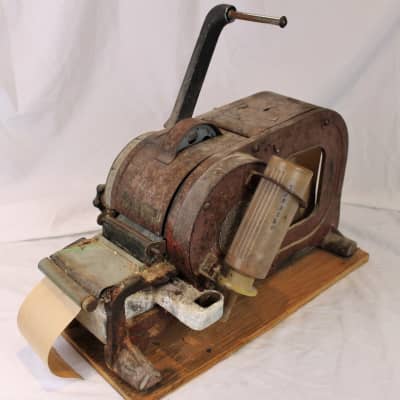The image depicts a vintage machine, possibly a tape shooter or another antique device used for tasks like printing or sewing. The machine, which has a rectangular, brown metal body with rusty patches, rests on a plain wooden plank. Mounted on a beige or white cloth background, it features complex mechanisms including rollers and a prominent black handle on the side. On the left side, there's an attached canister and a window, while tan-colored paper or tape protrudes from the front of the device. This well-used, outdated machine showcases intricate details and signs of age, offering a glimpse into past technology.